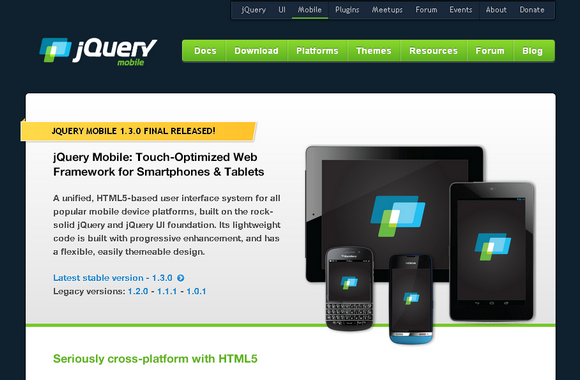This is a screenshot of a website dedicated to jQuery, a popular JavaScript library. The site has a navy blue background accented by a green navigation bar featuring tabs labeled "Docs," "Downloads," "Platforms," "Names," "Resources," "Forum," and more. Central to the page is a section with a white background showcasing various devices, including a Blackberry phone, a regular smartphone, a tablet, and a computer, to illustrate the diverse compatibility of jQuery.

The highlighted text prominently displays "jQuery Mobile" along with the tagline "Touch-Optimized Web Framework for Smartphones & Tablets," emphasizing the framework's optimization for mobile and touch devices. The latest stable version is mentioned in blue text, while legacy versions from 1.2.0, 1.1.1, to 1.0.1 are also listed. The website further asserts the framework's "Seriously Cross-Platform" capability with HTML5, underlining its broad applicability across different devices and platforms.